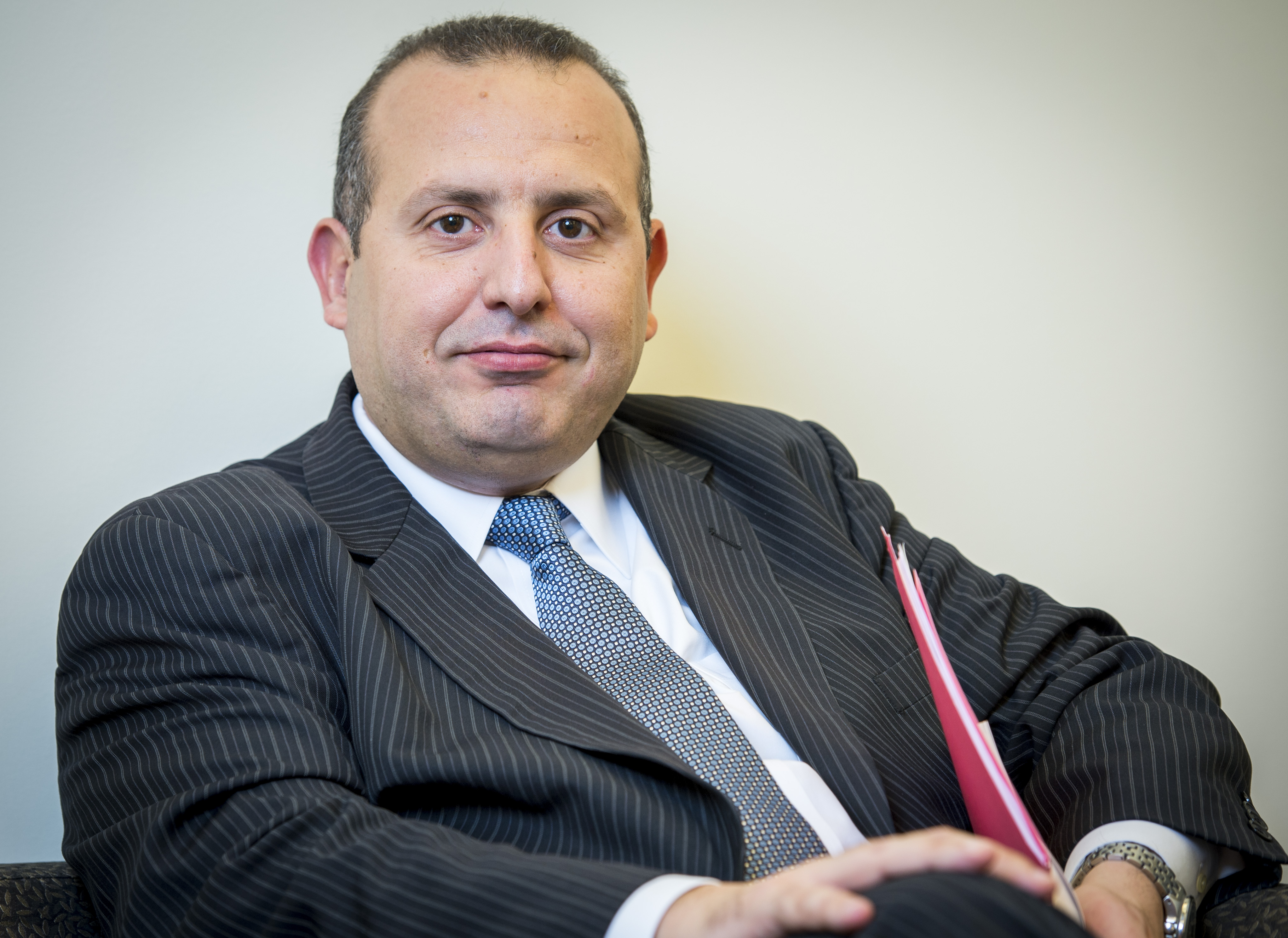The image features a slightly stout, Caucasian man with short buzz-cut brown hair and a receding hairline, predominantly visible above his forehead. He has dark brown eyes, slightly pointed eyebrows, and a faint smirk that lends him a relaxed demeanor. A light blue and gray pinstripe suit jacket envelops his upper body, paired with a white button-up shirt and a geometrically patterned blue tie, slightly askew as he sits angled towards the camera.

In the nook of his bent left arm, he clutches a red folder containing visible white papers, with his left hand resting on a surface that showcases a polished silver watch peeking out from his shirtsleeve. His right arm is casually placed on his knee, which is slightly raised. 

The backdrop is a light gray wall, with a subtle gradient brightening towards the man’s left side from the viewer’s perspective. Behind him, a small segment of a black chair is just visible at the lower left corner. The overall setting suggests an indoor professional environment, with the man's attire and overall pose indicating a formal portrait session.